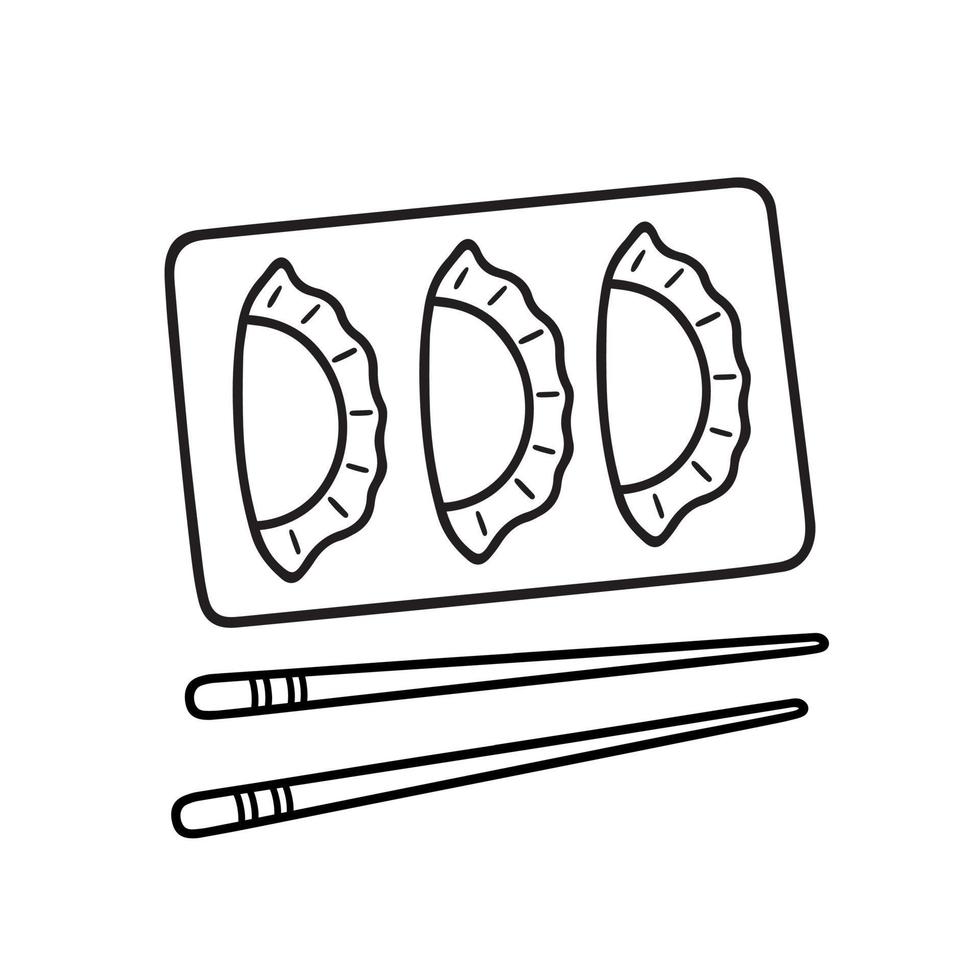In this simple yet detailed black-and-white line drawing, three Chinese dumplings are carefully arranged in a row on a slightly slanted rectangular plate. The long sides of the plate are parallel to the top and bottom edges of the image and are outlined with thick, black lines that suggest it might be a metal or wooden tray. Each dumpling is positioned with its flat side facing left and its scalloped, fluted edges pointing to the right, adding texture to the otherwise minimalist illustration. Below the plate, a pair of chopsticks, each adorned with two sets of horizontal lines near their thicker ends, are placed parallel to the bottom edge of the image. The tapered tips of the chopsticks and the overall lack of line variation, suggestive of a marker drawing, contribute to the illustration's straightforward and uncluttered style.